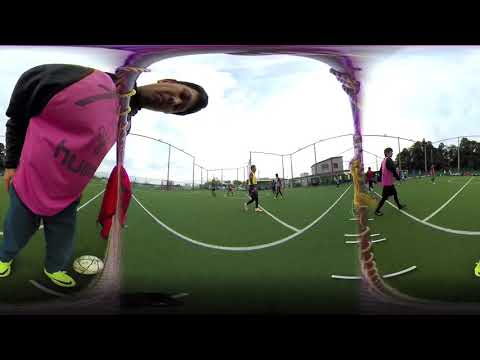In this vibrant, panoramic photograph taken outdoors on a soccer field, a man in a pink shirt with black sleeves and jeans is captured in three distorted sections, creating a surreal, fisheye effect. The man, who has short dark hair and a darker complexion, is positioned on the left side, leaning and looking sideways towards the center of the image. A white soccer ball lies near his bright green sneakers at the bottom. The field, marked with white lines, stretches out under a bright blue sky dotted with white clouds. In the distance, players in yellow, pink, and red jerseys are dispersed across the field, with tall fencing and some trees outlining the horizon. This panoramic shot, stylized with photographic representationalism, merges different perspectives, including an unusual, oversized depiction of the man, adding an abstract, almost surreal quality to the scene.